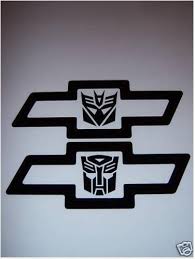The image features a white background with a small, indiscernible logo situated in the bottom right corner. At the center, there are two skewed plus-shaped objects in a black or dark gray color, each containing a stylized face. The plus shapes tilt slightly to the left. The top object depicts a woman's face, while the bottom object shows a man's face. The design bears some resemblance to the cross-like shape of the Chevrolet logo, and the faces evoke an ancient or mythological aesthetic, potentially reminiscent of Sumerian or Tartarian deities. The overall graphical rendering combines minimalist elements with a subtle use of gray tones, possibly with a hint of blue.